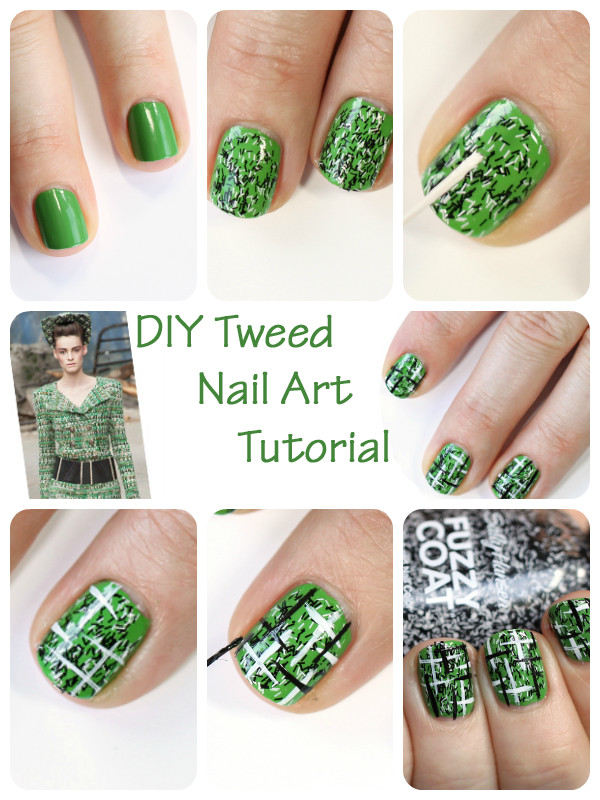This is a vertical rectangular image designed as a cover for a nail art tutorial booklet or website. The centerpiece features green text reading "DIY Tweed Nail Art Tutorial." Surrounding the text are eight photographs showcasing various stages and styles of tweed-inspired nail designs, predominantly in green, black, and white hues. 

- **Top left**: Two fingers with solid green painted nails.
- **Second from the left on the top row**: The same fingers with additional short green, black, and white lines creating a textured appearance.
- **Third from the left on the top row**: The same nails with a tool being used to poke and refine the tweed pattern.
- **Top right**: A close-up of three fingers exhibiting intricate white patterns over green nails, resembling tweed.
- **Bottom left**: Another set of fingers with varying green and white lines forming a tweed-like texture.
- **Second from the left on the bottom row**: A woman's nails showcasing the final tweed design in green, black, and white, with the woman's tweed jacket in the background, mirroring the nail pattern.
- **Third from the left on the bottom row**: A different angle of the green and white patterned nails with black specks.
- **Bottom right**: A close-up of nails with the completed tweed design.

The background has a cohesive green theme that ties all the images together, and the inclusion of a woman in a matching tweed jacket reinforces the tutorial's focus on achieving this stylish look.